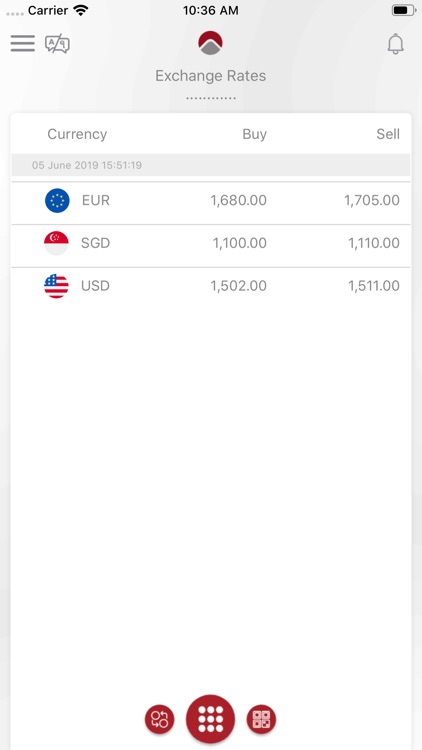In the image, we see a snapshot of a financial data website from Carrier, timestamped at 10:36 AM. The display indicates a battery level at about 70% charged. Central to the screen are exchange rates, prominently featured with a gray and maroon emblem above them. Down the left side, various currencies are listed, each accompanied by corresponding buy and sell prices.

The header reads "05 June 2019, 15:51.19," indicating the date and precise time. The first listed currency is EUR (Euros), symbolized by a red circle with stars around it, representing the European Union countries. The exchange rate for buying Euros is 1,680.00, while the selling price is 1,705.00. 

Next, SGD (Singapore Dollars) is represented by a flag featuring a red semicircle at the top with a crescent moon and five stars, and a white lower half. The buy price for SGD is 1,100.00, and the sell price is 1,110.00.

Following that is USD (US Dollars), represented by an American flag with red and white stripes and a blue field with white stars. The buy rate for USD is 1,502.00, and the sell rate is 1,511.00.

At the bottom of the screen are several icons. Central is a prominent red oval encasing a 3 by 3 grid of white circles. To the left, an oval icon features two holes with arrows forming a circular pattern between them. To the right, another oval displays four white boxes with dots, resembling dice: the upper left, upper right, and lower left boxes each have one dot, whereas the lower right box has two dots.